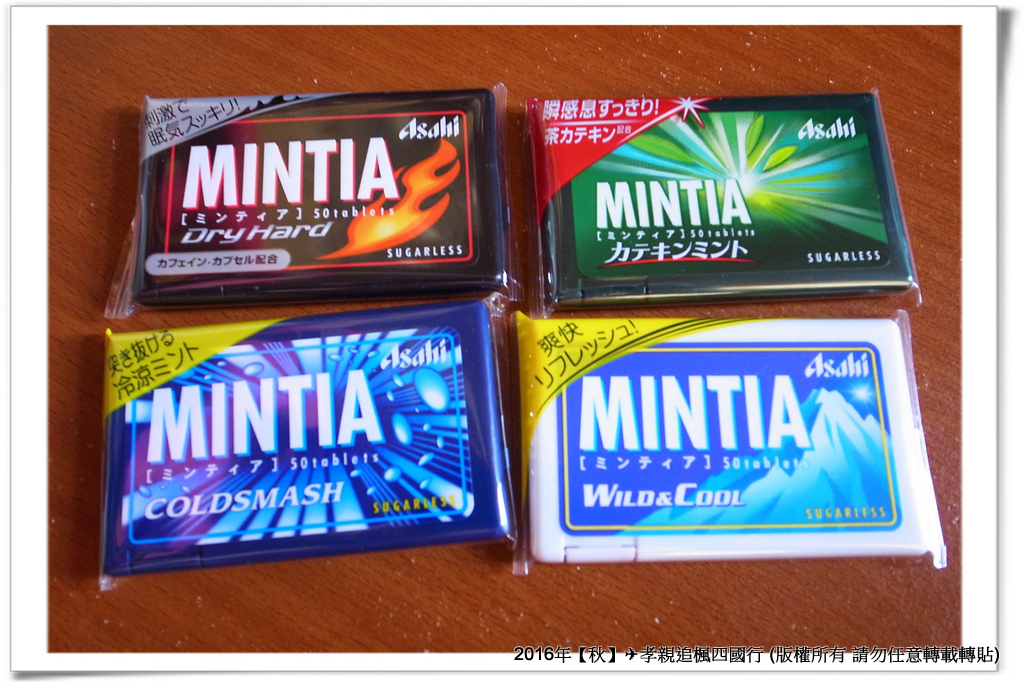The image depicts four packages of Mintia mints, each sealed in cellophane and arranged on a reddish-brown wood grain table. The packages, made by Asahi, feature different vibrant colors and designs to denote various flavors. The top left package is black with a flame design, labeled "dry hard." Below it, on the bottom left, is a dark blue package with radiating blue splash marks, labeled "cold smash." Adjacent to the dark blue pack, the bottom right package is white with an image of a snow-capped mountain peak, labeled "wild and cool." Finally, the top right package is green with a starburst pattern and some leaves, labeled in an Asian language. All packages are sugarless and prominently display the Mintia brand name at the bottom center with Asahi written in cursive at the top right. The table's wood grain slants at about a 45-degree angle in the photograph.